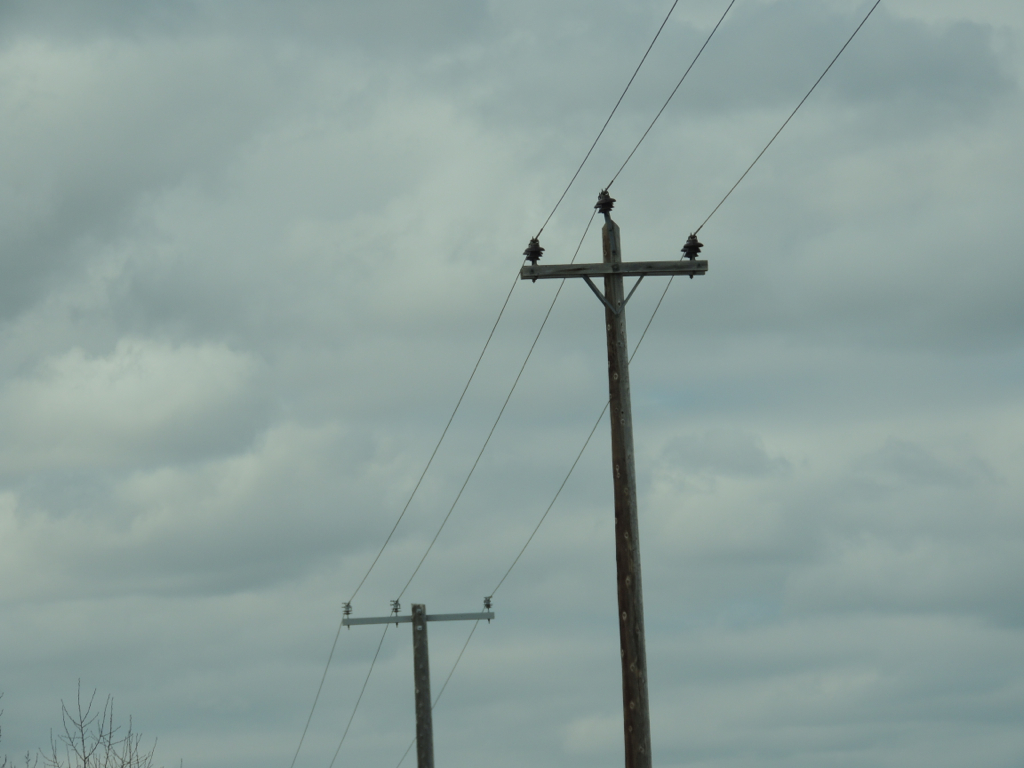This dimly lit photograph features two weathered, large wooden telephone poles each with a single wooden crossbar near the top, supporting a total of three power lines. These lines stretch horizontally across the frame, eventually disappearing off the edges of the image. The background is dominated by an overcast, mostly cloudy sky, creating a mood of gray monotony with minimal color variation. In the lower left-hand corner, there is a glimpse of a leafless tree with skeletal branches, adding to the somber and desolate atmosphere of the scene. The photograph is devoid of any text or other descriptions.